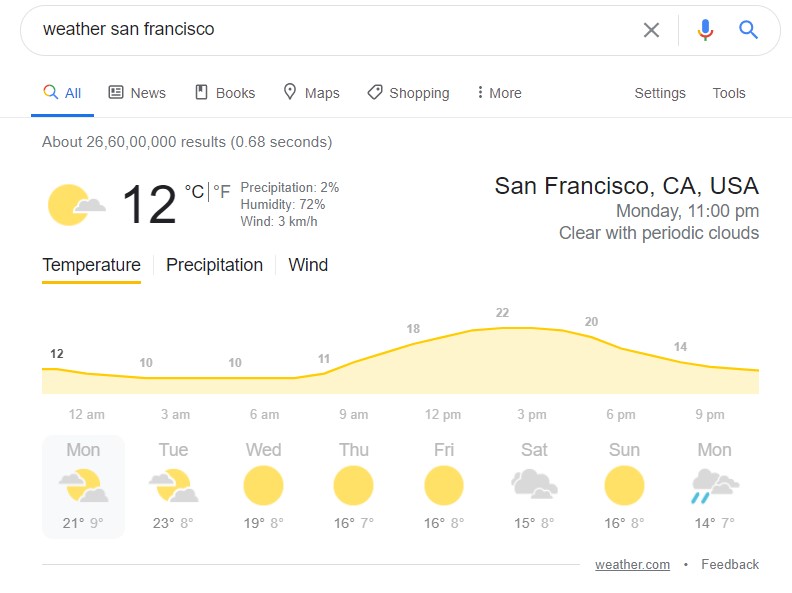The image is a detailed screenshot of a weather search result for San Francisco, California on Google. At the top, the search box displays "weather San Francisco." Just below the search box, there are horizontal labels including All (highlighted in blue), News, Books, Maps, Shopping, More, Settings, and Tools. The search result yields approximately 2,660,000,000 results in 0.68 seconds.

Prominently displayed is a weather icon with a sun partially obscured by a gray cloud, indicating the current weather condition. The temperature is shown as 12 degrees Celsius (54 degrees Fahrenheit), with additional details of 2% precipitation, 72% humidity, and a wind speed of 3 kilometers per hour. To the right, it specifies the location as San Francisco, California, USA, with a time stamp of Monday, 11 p.m., noting the weather as "clear with periodic clouds."

Below this main section, three more tabs are provided: Temperature (underlined in orange), Precipitation, and Wind, accompanied by a horizontal line illustrating the weather trend. Further down, an eight-day weather forecast is presented with the following temperatures:

- Monday: 21°C
- Tuesday: 23°C
- Wednesday: 19°C
- Thursday: 16°C
- Friday: 16°C
- Saturday: 15°C
- Sunday: 16°C
- Monday: 14°C

The forecast for the upcoming Monday includes an icon indicating rain and heavy clouds. At the bottom of the screenshot, there is a reference to "weather.com" and an option for feedback, with no other text visible. This image results from a search query for the weather in San Francisco, California.